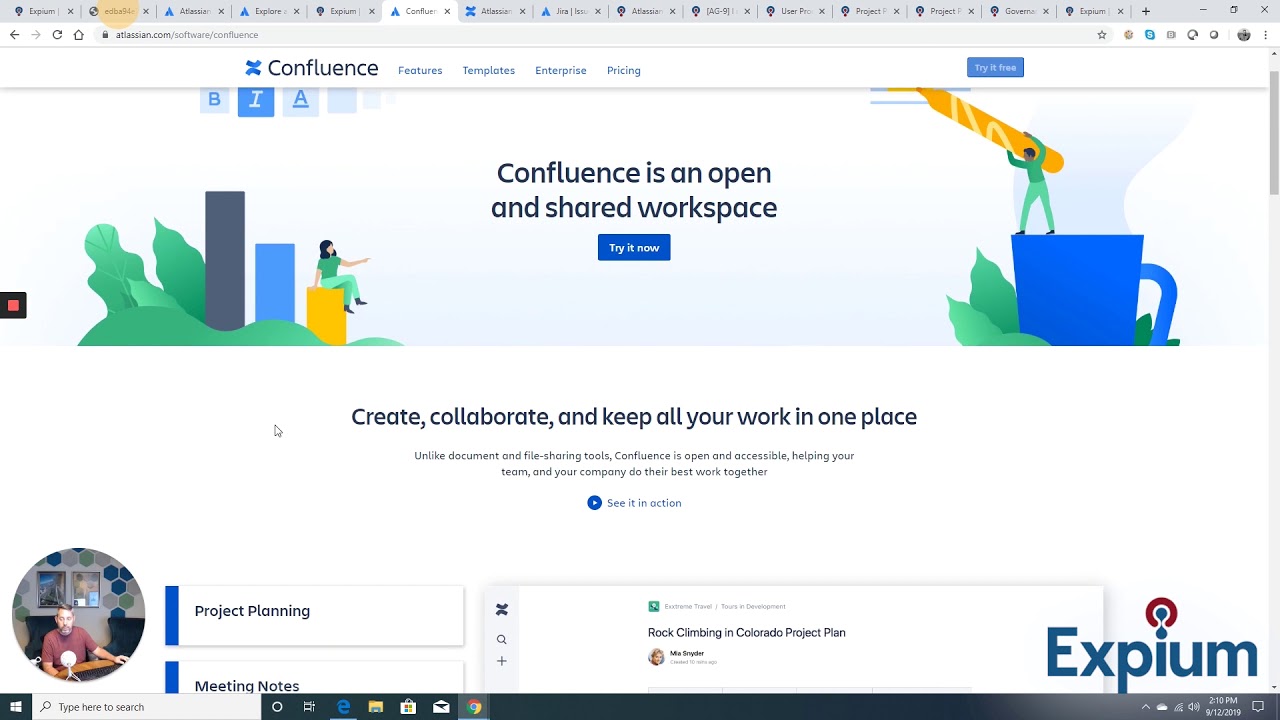A screen capture of a Google Chrome browser displays a window with around 15 to 20 open tabs. The active tab is showcasing the Confluence website, which promotes itself as "an open and shared workspace." The page features animated cartoon illustrations, including a person sitting on a yellow bar of a bar graph, with a blue bar and a purple bar in the background. Another cartoon figure is depicted standing on a blue coffee mug, using a pen or pencil to draw something. The website encourages users to "create, collaborate, and keep all your work in one place," and highlights functionalities such as project planning and meeting notes. An avatar picture is also visible, reinforcing the collaborative nature of the platform. The call-to-action "Try it now" is prominently displayed, inviting users to experience the Confluence workspace.